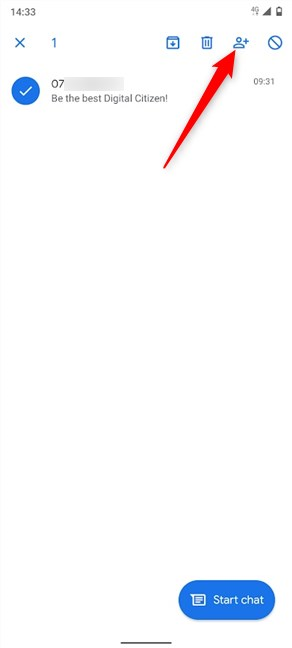The image features a white background with several user interface elements. In the top right corner, there are icons displaying the signal strength and a battery level at approximately 25%. On the top left, the time reads 14:33. Below the time, there is a blue "X" icon followed by a blue "1."

To the right of these elements, there is a small box with a downward-pointing arrow, followed by various icons: a trash can, a figure of a person accompanied by a star, and a circle with a diagonal line through it. A prominent red arrow points directly at the icon of the person with a star.

Further down the image, there is a blue circle with a white checkmark inside it. Next to this circle is a partially blurred segment displaying "07," though the ensuing text is obscured. Additionally, the time "09:31" is visible, along with the text "Be the best digital citizen."

At the bottom of the image is an oblong dark blue button featuring a text bubble icon with the label "Start Chat." Below this button, to the left, runs a thin black horizontal line.